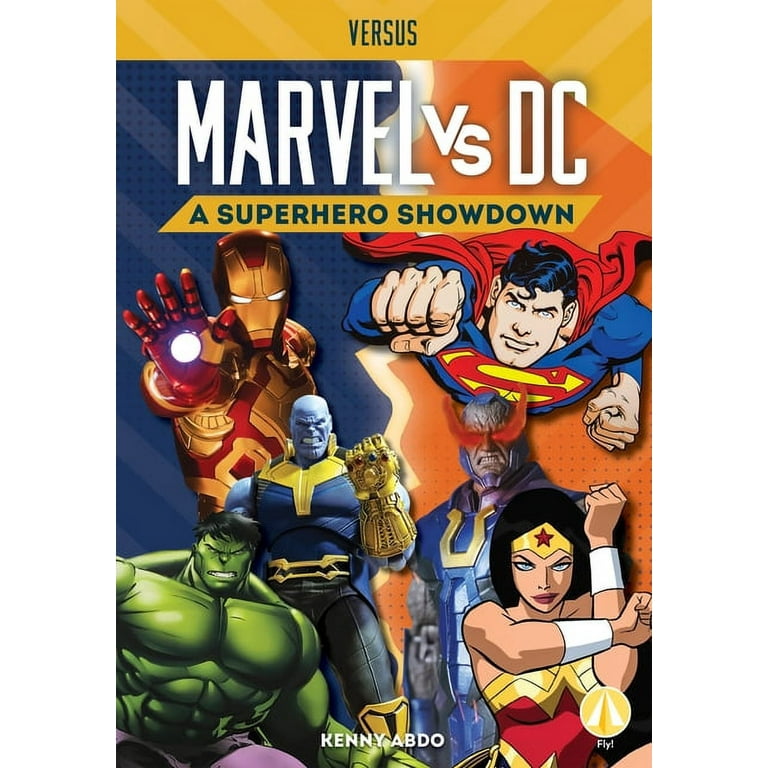The comic book cover titled "Marvel vs DC: A Superhero Showdown" showcases an epic battle between iconic superheroes from both universes. At the top, the word "VERSUS" is prominently displayed, followed by "Marvel vs DC" in bold white letters, and "A Superhero Showdown" underneath in smaller blue letters on a yellow banner. The bottom of the cover credits Kenny Abdu. The left side of the cover, tinted in blue, features DC characters Superman and Wonder Woman, illustrated in a classic cartoony comic style. In the center of them appears a villain in a realistic CGI style, enhancing the contrast. The right side, glowing in orange, portrays Marvel characters Iron Man, rendered with cartoony details, the Hulk in a realistically shaded comic book drawing, and Thanos with his iconic Infinity Gauntlet in a hyper-realistic CGI design. The heroes and villains are dynamically arranged with overlapping positions, creating a sense of depth and motion. A striking lightning bolt divides the composition, symbolizing the intense clash between the two universes. The characters dominate three-fourths of the cover, ensuring an action-packed visual experience.